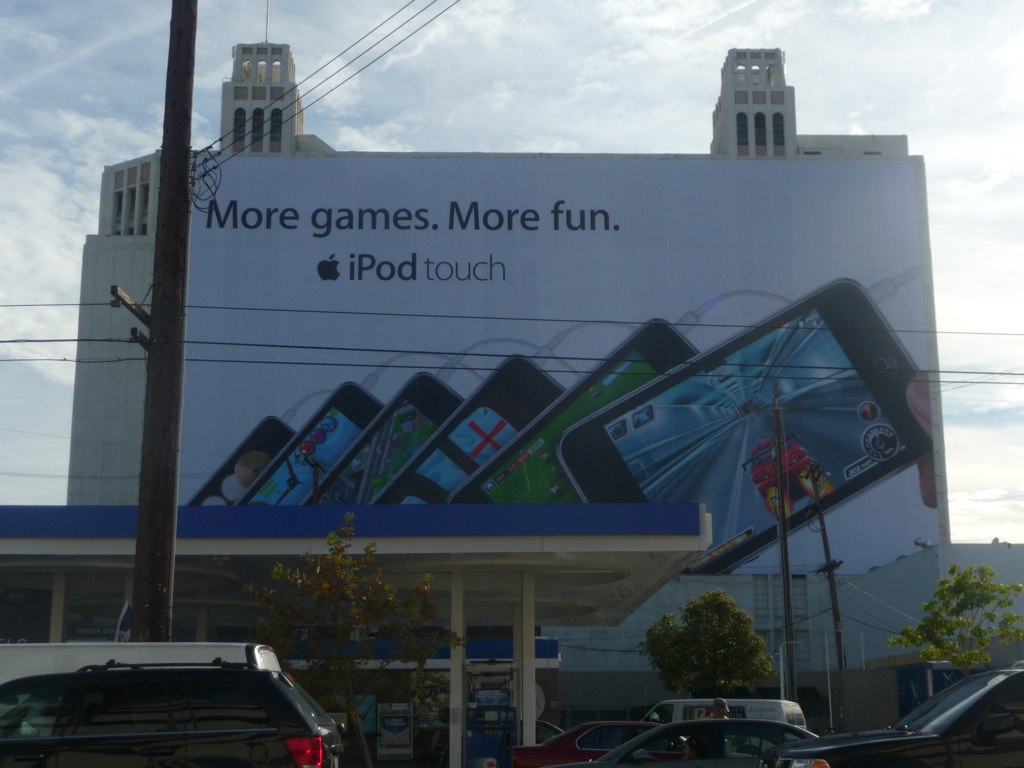In this urban scene, a large photograph captures the bustling activity around a gas station set against the backdrop of a prominent building. The side of this building showcases a massive Apple advertisement for the iPod Touch. The billboard, characterized by its clean white background and bold black text, reads "More Games, More Fun," punctuated by the iconic Apple logo and the words "iPod touch." Below the tagline, several iPod Touch devices are displayed in a row, each screen featuring different games. The gas station in the foreground has a distinct blue and white awning supported by white columns and a white ceiling. Several parked cars and a white van are visible, with trees interspersed throughout and a few telephone pole wires and a pole at the image’s left edge. The image captures a sense of everyday urban life, with a person standing outside a car and another driving by, all within the shadow of the towering building that features two tower-like structures atop it.